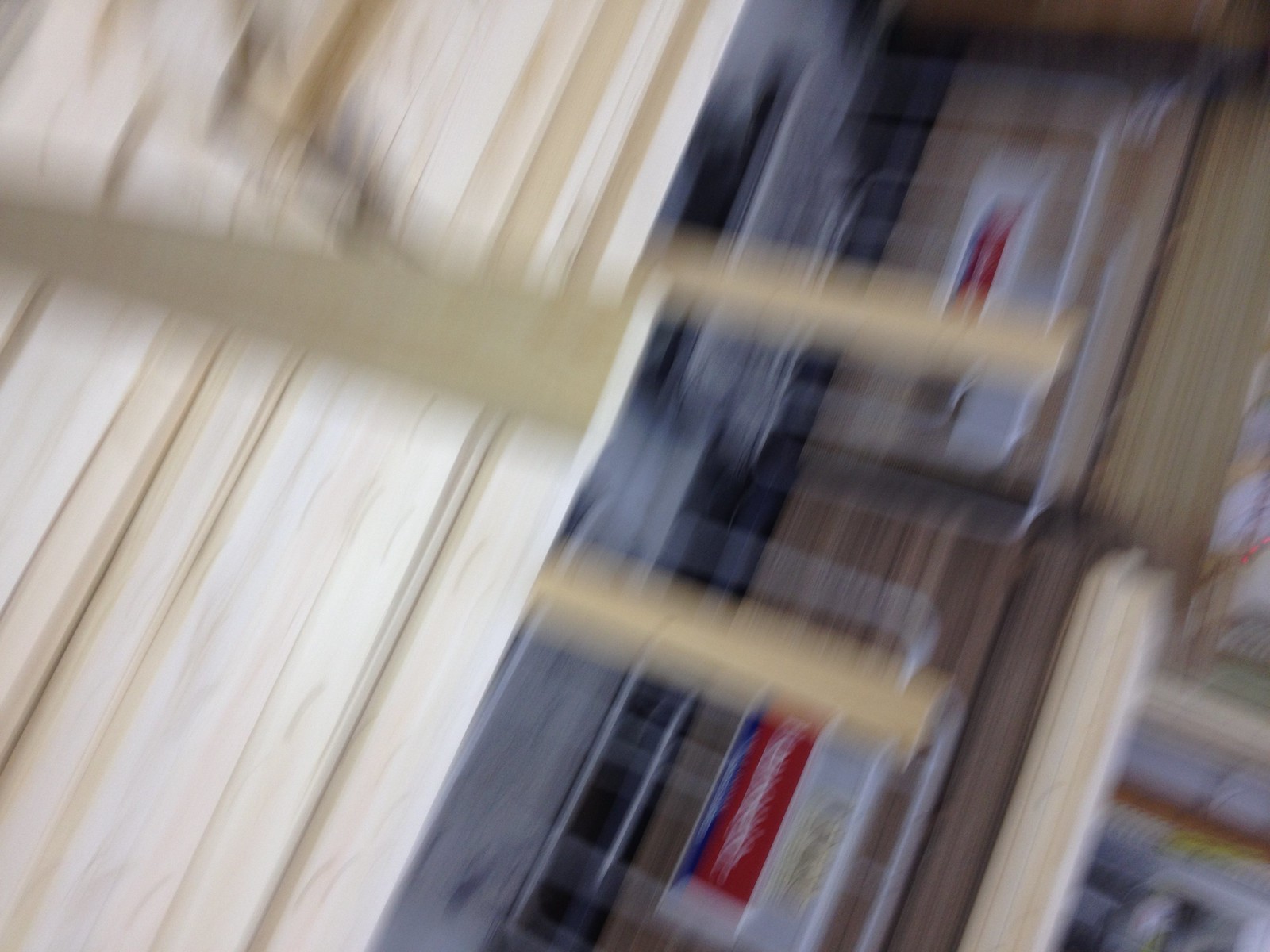A highly blurry image depicting what appears to be an assortment of indistinguishable objects, possibly boxes, with various shades of brown, white, and black. The extreme blurriness creates a sense of confusion and makes it impossible to identify specific details. The angle suggests it was accidentally taken at hip height, perhaps as the photographer was removing their phone from their pocket, resulting in this unintentionally captured moment.